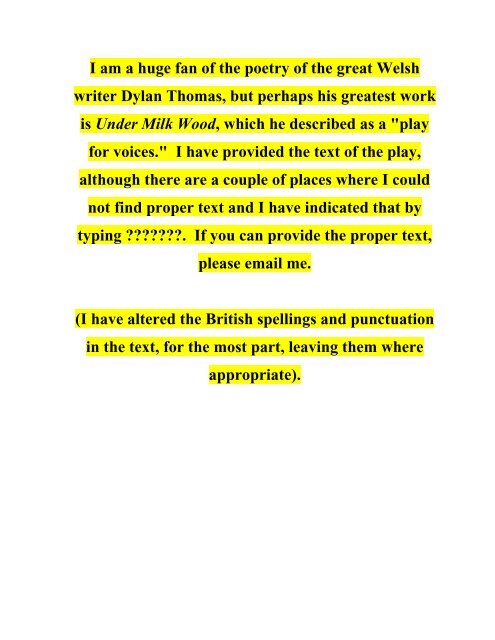The image depicts a section of text against a white background. The text, written in black, is highlighted in yellow, which makes it stand out prominently. The content of the text reads: "I am a huge fan of the poetry of the great Welsh writer Dylan Thomas, but perhaps his greatest work is *Under Milkwood*, which he described as a play for voices. I have provided the text of the play, although there are a couple of places where I could not find proper text, and I have indicated that by typing '??????' (repeated six or seven times). If you can provide the proper text, please email me. I have altered the British spellings and punctuation in the text for the most part, leaving them where appropriate." The cohesive design of the text against the white background, highlighted in yellow, ensures clarity and readability.